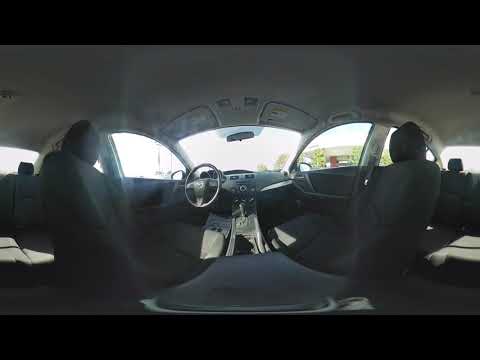The image shows the interior of an empty vehicle, viewed from the backseat. The car's interior predominantly features dark gray and black tones, with the seats, dashboard, and steering wheel all in black. The ceiling liner and visors are a light gray. The image appears distorted with the front seats placed at an odd angle, almost sideways, creating a warped effect. 

Both the driver's side and passenger's side are devoid of any passengers or personal belongings, giving the car an abandoned or isolated appearance. Despite the clear daylight outside, visibility through the windows is minimal due to a blown-out effect, leaving the main view dominated by white, with hints of green trees and possibly a gray building outside. Additionally, the image includes black bars at the top and bottom, framing the scene.